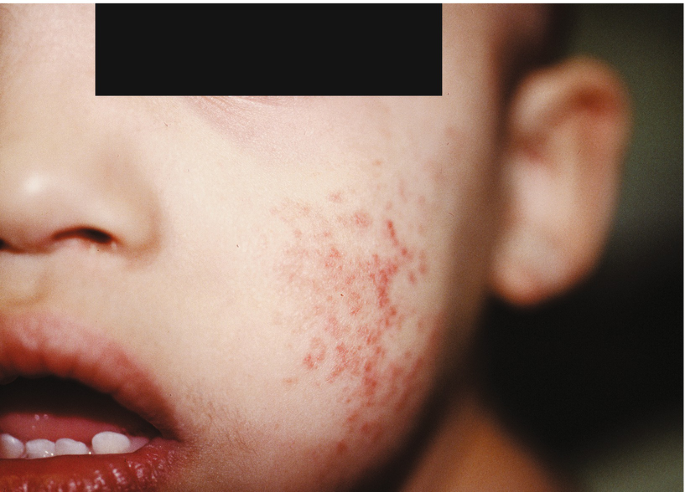This is an extreme close-up medical image of an infant's face, predominantly focusing on the left side. The child's eyes are obscured by a black bar to protect their identity, giving the image a clinical or medical textbook appearance. The infant's mouth is wide open, revealing four small teeth and a visible tongue. The lips appear cracked and dried, suggesting dehydration, and there are crusty residues around the mouth and nose. The cheek is noticeably afflicted with a splotchy, red rash that covers a significant area. The background shows a blurred ear and neck, emphasizing that the main focus is on the facial rash. The overall image evokes concern due to the child's distressed appearance, possibly indicating illness, such as a fever or a skin condition.